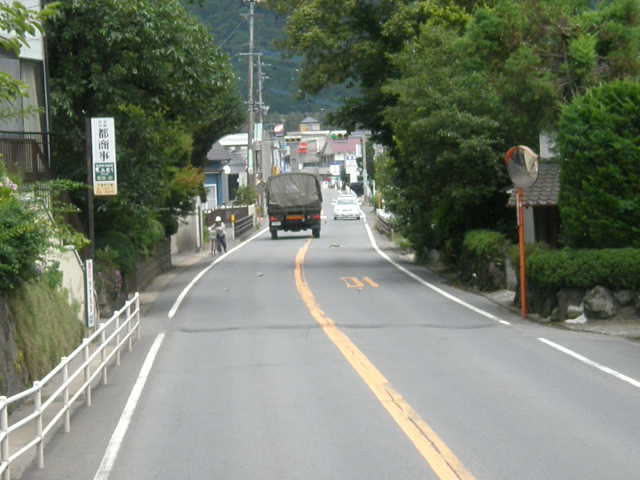The image depicts a narrow, two-lane road in Japan with a distinct yellow dividing line and narrow shoulders. On the right side, there's an abundance of trees, some arching over the road, while the left side features additional foliage, a white railing, and a green and white street sign with Japanese symbols. In the foreground, a person is pushing a bicycle towards the viewer. Alongside them, there's a mirror mounted on a pole for traffic navigation and an orange pole nearby. The road briefly descends towards a small town, identifiable by modestly sized buildings and a congested layout typical of urban Japan. Two vehicles are visible: a white sedan approaching and a fabric-covered truck heading away. The scene includes power lines, traffic lights, and an entryway cut through shrubs leading to a building with a brown roof. In the far distance, there's a mountainous backdrop completing the picturesque landscape.